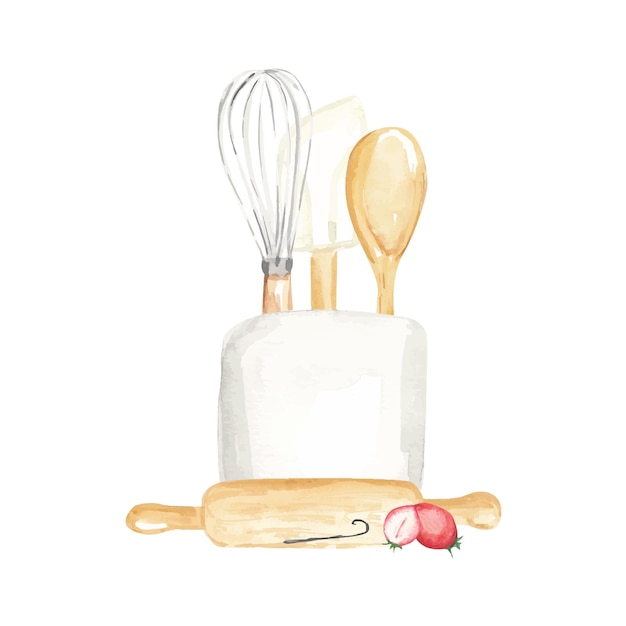The image appears to be an artistic drawing of a kitchen scene. Central to the composition is a white canister holding three baking utensils: a silver whisk with a tan handle, a white spatula with a tan handle, and a tan wooden spoon. In front of the canister, on the ground, lies a tan rolling pin with a black hook on its side. Adjacent to the rolling pin are two halved strawberries, showcasing their red interior, seeds, and hints of green leaves. The background of the image is entirely white, giving a clean and minimalistic feel to the scene. The drawing is lightly colored, focusing primarily on shades of brown, white, and the metallic sheen of the whisk.